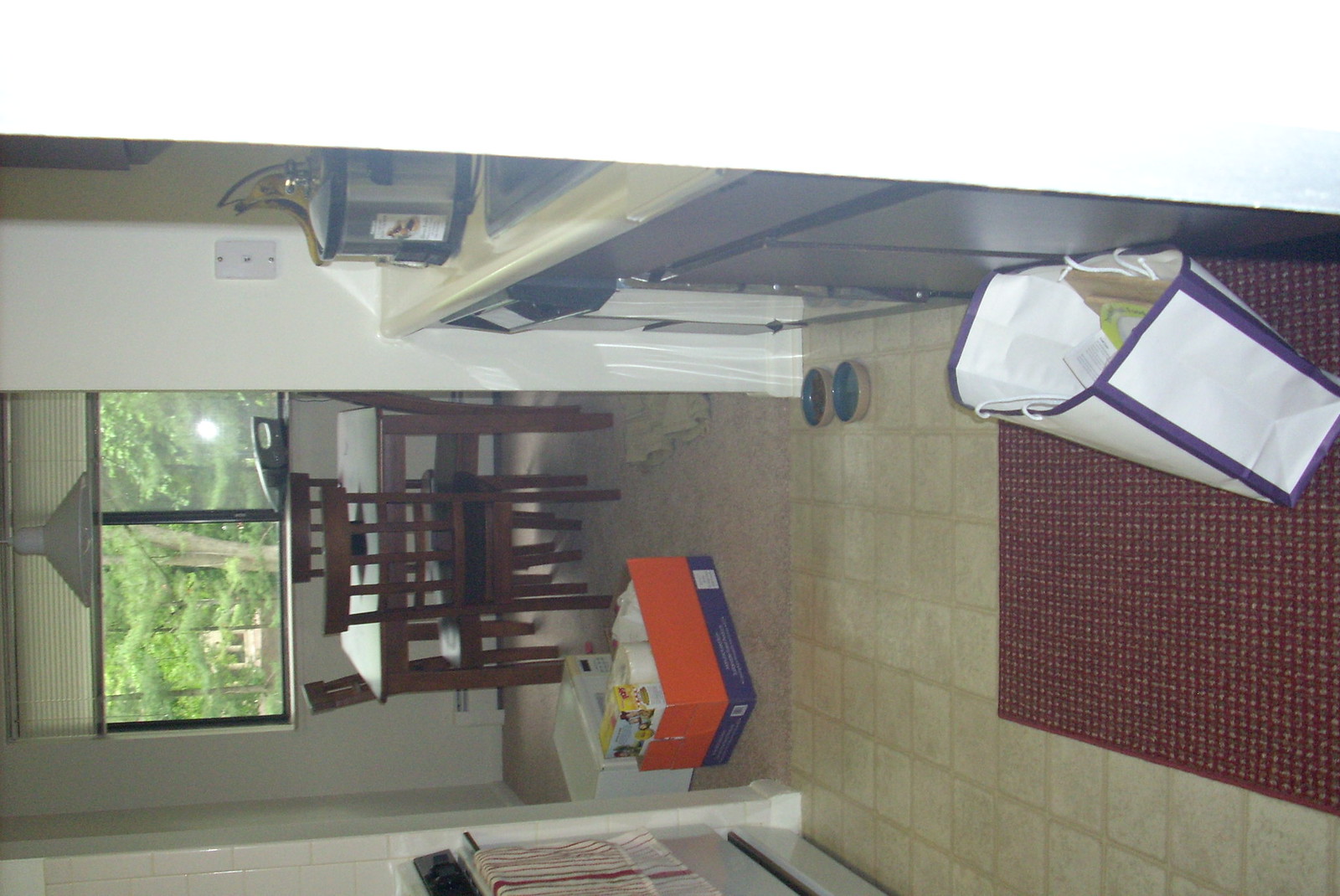This photograph, which was taken sideways, captures a cozy interior of a home focused on a small galley kitchen. The kitchen has a light brown linoleum or vinyl floor that mimics the look of tile, with a red rug positioned in front of the sink. On the rug rests a white and blue tote bag, its contents obscured. The cabinets are a distinctive blue-gray, complementing the off-white countertops. A glass jug sits on the counter, and a stove with a towel draped over the oven handle is visible on the opposite side.

Beyond the kitchen, through a doorway, lies another room. There, you can see an orange box with a blue lid filled with various items, such as paper towels and possibly a box of cereal. Behind this box, a white appliance, likely a microwave, rests on the floor.

In this adjoining room, a square table with four chairs is set up near a window. Outside the window, green trees with lush leaves and the silhouette of another house are visible. A small vacuum appears to be situated on the windowsill, which is partially covered by a white shade pulled up to about one-fourth of the window's height. A light fixture hangs from the ceiling over the dining area. Additionally, two pet bowls are placed on the kitchen floor, suggesting the presence of a pet in the home.